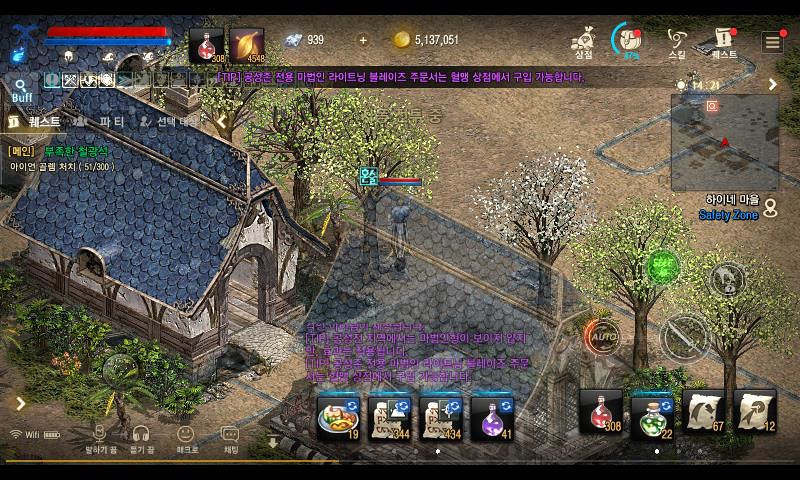This detailed screenshot from a video game captures a rich medieval setting. Dominating the left side of the image is a medieval-style building reminiscent of a hobbit's abode, constructed with white tan stone walls and dark, ornate wooden arcs. The gray slate roof, peppered with rounded shingles resembling scales, features a prominent dormer and an arched window. The heavy lumber-framed, diagonally facing front door adds to the authenticity, and a lush garden or foliage enhances the scene to the left. 

To the right, a vast tan field extends across the top and down the side of the image, interspersed with animated trees, including one with distinctive white leaves. At the bottom, eight icons are displayed, likely representing weapons, powers, and potions, each accompanied by various numerical values. The top of the image is a dense repository of game stats and information, including a map in the upper right corner marking the player's position with a red dot.

Additional details include a dark brown background on the top left featuring a straight red line above a solid blue line, likely indicating some status metrics. In-game currency and resources are also visible, such as a gold circular coin (5,137,051) and a diamond icon (939). The interface and text appear to be in either Chinese or Japanese, contextualizing the game's origin. Moreover, a pair of headphones and emotive circles (smile/unhappy) are noted by the score information on the left.